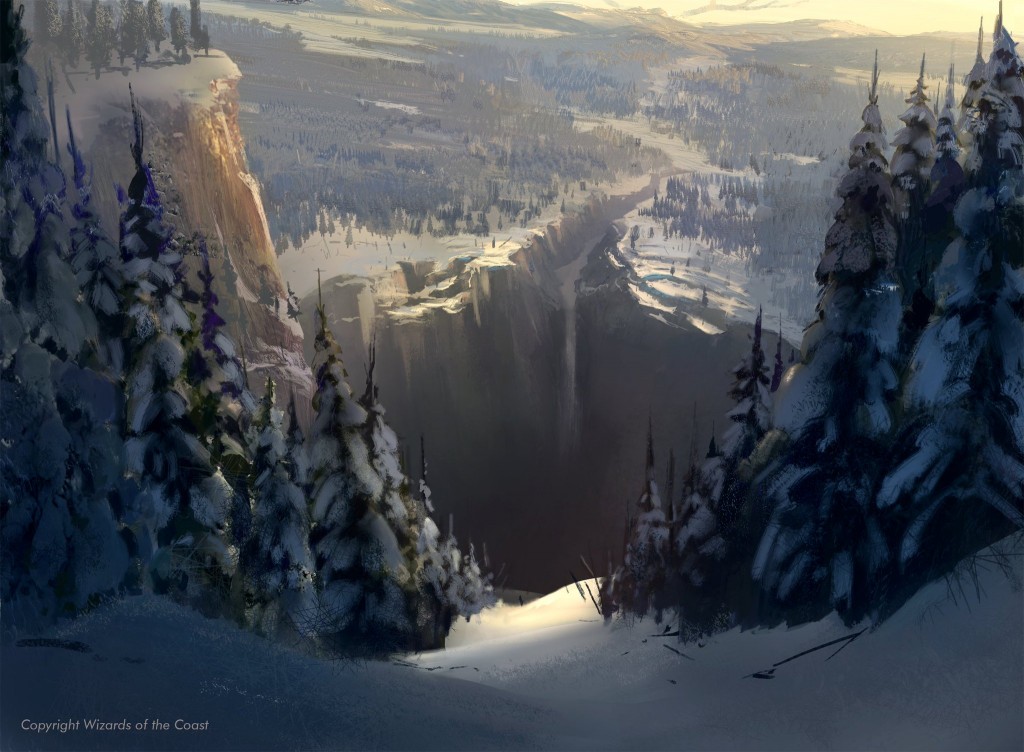This painting captures a breathtaking winter landscape, portraying a snow-covered ridgeline that leads to a dramatic drop-off into a vast ravine. The ridgeline is adorned with snow-laden evergreen trees, with those on the left showing unique purple tips while those on the right have pristine white tips. As the terrain descends into the cliff edge, the imposing brown cliffs mark the entrance to a large ravine. Flanking this ravine, a dense forest of snow-capped trees extends far into the distance, creating a deep, snowy valley.

At the forefront of the painting, a snowy path leads into the scene, inviting viewers to explore further. Larger, more detailed pine trees frame this path, enhancing the illusion of standing between these towering giants. The scene is enveloped in an ambient light with a hint of yellow sky on the right side, suggesting an early or overcast day. The background features lofty, snow-draped mountains, adding majesty to the composition. Additionally, there’s a clearing on the left side that may hint at a snowy field or perhaps a distant body of water.

The overall palette comprises whites, dark greens nearly black under the snow's weight, and the earthy browns of the sheer cliff faces where the snowfall breaks. As a finishing touch, the painting holds a subtle acknowledgment of its creation: the bottom left corner bears a copyright by Wizards of the Coast. The combination of intricate details and expansive views makes this painting a striking depiction of a serene and imposing winter wilderness.